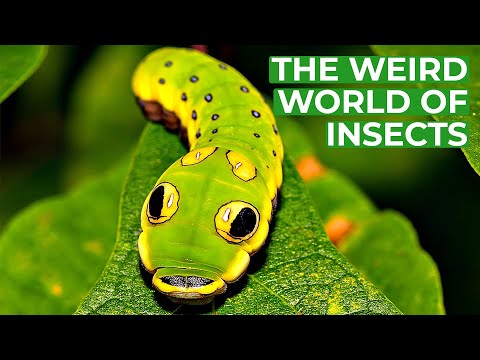The image is a close-up of a caterpillar, prominently featured against the backdrop of a leaf. It appears to be a highly detailed illustration or a photograph, possibly gracing the cover of a nature-themed publication such as Ranger Rick or National Geographic, under the title "The Weird World of Insects." The caterpillar itself is strikingly vivid, showcasing a bright lime green body with bold lemon yellow edges and spots. Most notably, it has large, black "eye spots" on its rear that are surrounded by vibrant yellow, mimicking the appearance of a face to deter predators. Its segmented body is meticulously detailed, with tiny black polka dots encircled by white, and yellow stripes running along its underside, possibly hinting at legs. The insect sits on a dark green leaf, where the intricate veins are clearly visible, while the background is filled with additional muted leaves, accentuating the foreground subject.